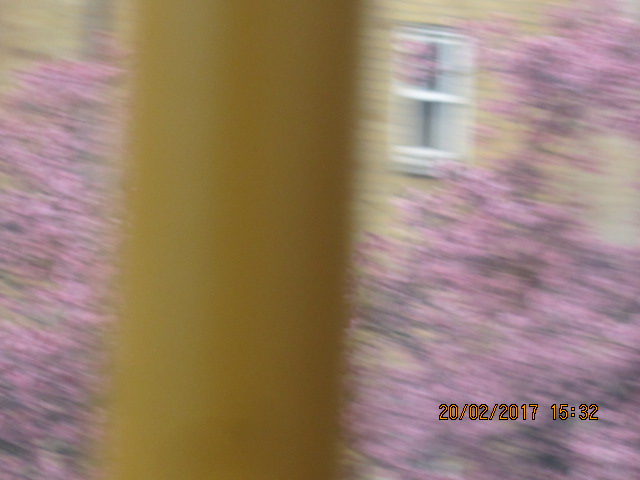This photograph, despite its significant blurriness and apparent camera shake, depicts the exterior of a house. The house has a tan or light brown brick wall with a white-framed window situated in the upper right area. In the foreground, thick clusters of pink flowers, which might be part of a pink tree or bushes, dominate the scene, creating a vivid barrier between the house and the camera. A yellow vertical shape, perhaps a pole or a rectangular object, stands prominently slightly left of the center, cutting through the floral display. The image includes a timestamp in the bottom right corner, reading "20-02-2017, 15:32" in yellow text, indicating the photo was taken on February 20, 2017, at 3:32 PM.